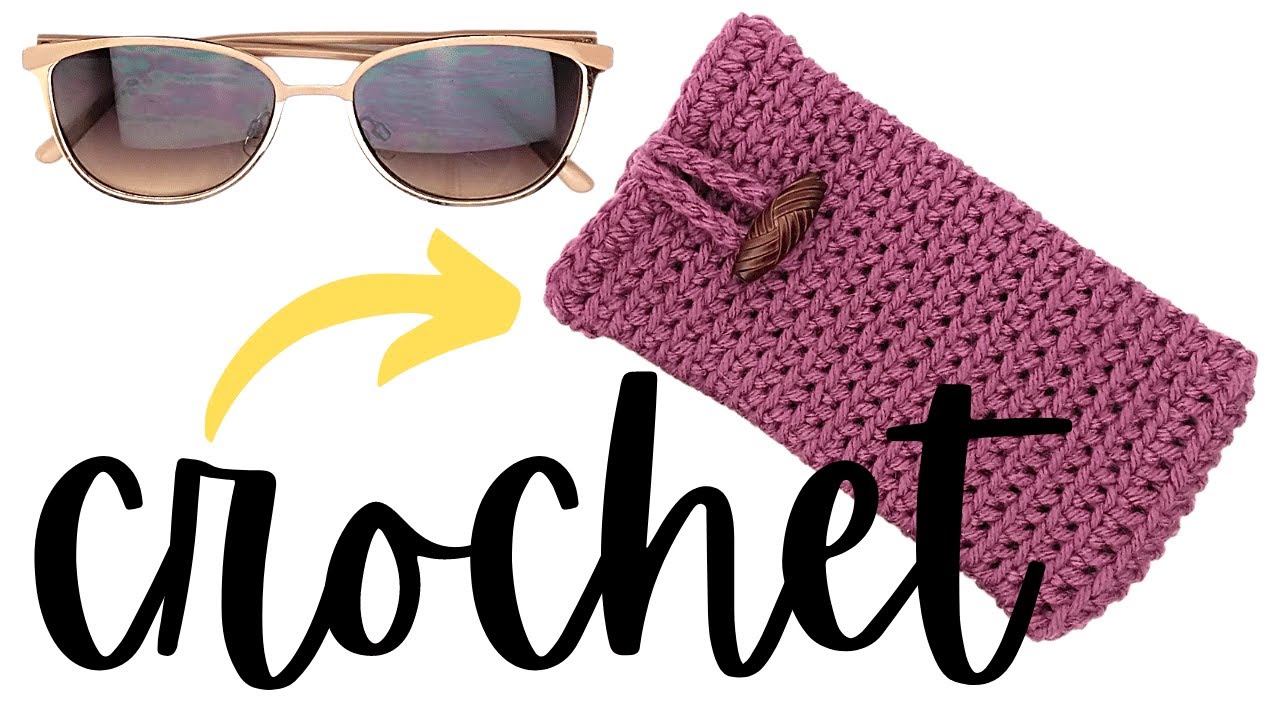This photograph features a pair of vintage-style sunglasses with dark brown, tinted lenses and a rose gold, horn-rimmed frame. The sunglasses are folded and situated in the upper left portion of the image. Below the sunglasses, in large, bold, black cursive script, the word "crochet" is prominently displayed. Just above the "R" in "crochet," a curved yellow arrow points to the right, directing attention to a crocheted glasses case. This case is made of mauve pink yarn, with a distinctive oblong brown button. The case is displayed at a diagonal tilt from the bottom right-hand corner towards the top center. Above the arrow and to the left of the case, the folded sunglasses and the crochet case present a harmonious composition, accentuated by a background featuring a piece of paper with pink, teal, and white wave patterns. No people or specific locations are indicated in the photograph, keeping the focus entirely on the stylish sunglasses and the intricately designed glasses case.